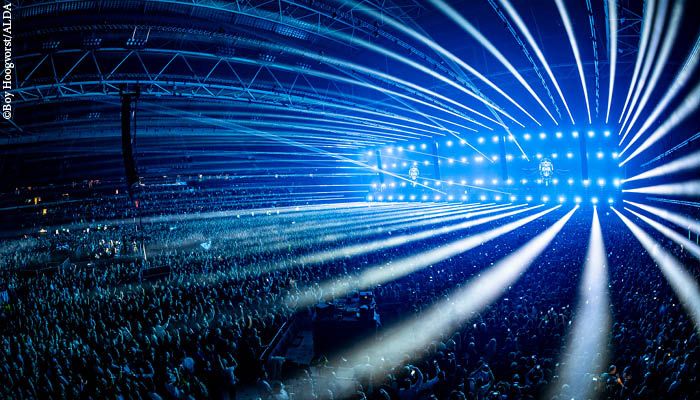The image, taken from a high vantage point at a concert, captures an expansive view of the venue filled with tens of thousands of attendees. The scene is bathed in a blue hue from the ambient lighting, creating a dramatic atmosphere. Two large screens dominate the background, each displaying an image of the artist, with bright lights radiating from the screens and forming vivid streaks that extend towards the camera. The light reflections and laser show add to the electric ambiance, with numerous white lights shining into the audience. Above the crowd, a network of metal bars and a rafter system can be seen, one of which supports a camera filming the event. In the midst of the crowd, the faint outline of a sound booth is visible, indicative of the behind-the-scenes efforts to elevate the concert experience.